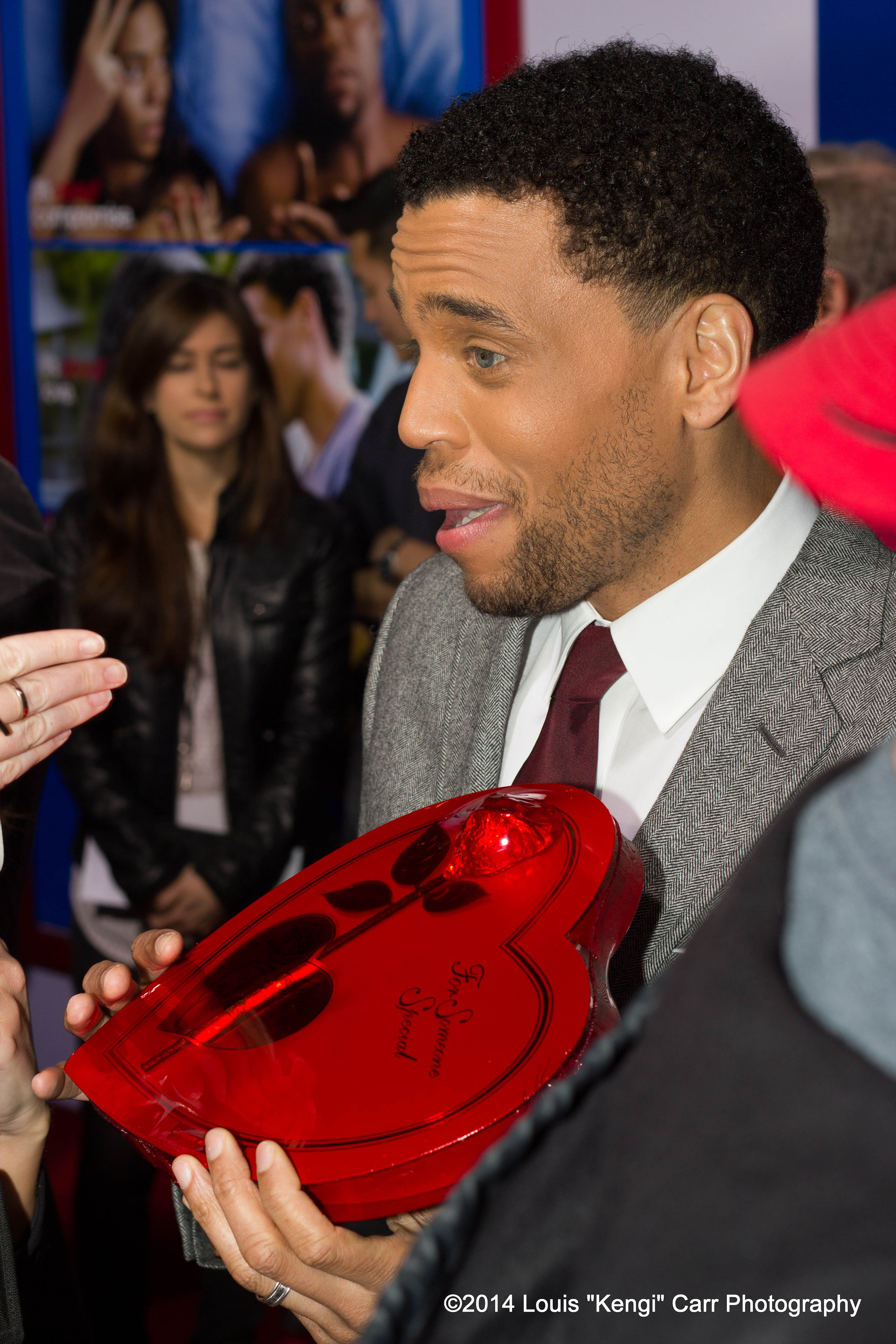Set against a backdrop that suggests an event or a gathering, the focal point of this image is a man positioned centrally, facing slightly to the left. The background features several people and what appears to be photographs or artwork adorning the walls. The man, an African American with short black hair, a stubbly beard, and mustache, gazes to the left with an expression of mild surprise and a hint of a smile. His striking hazel eyes add a touch of warmth to his demeanor. He is elegantly dressed in a black and white suit paired with a white collared shirt and a maroon tie. Prominently displayed in his hands is a large, red, heart-shaped box of Valentine's Day chocolates, adorned with a rose and labeled "For Someone Special." A hand, with just the fingers visible, likely belonging to someone handing him the box, can be seen on the left side of the image. This photograph, credited to Louie "Ken Gee" Car Photography from 2014, seems to capture a moment of genuine emotion and surprise amidst a social gathering.